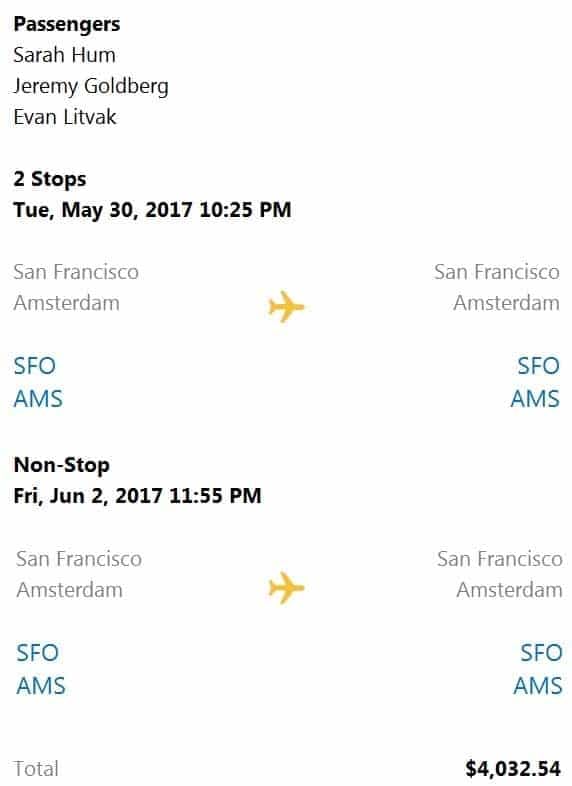Screenshot of a trip itinerary for passengers Sarah Hum, Jeremy Goldberg, and Evan Litvak. The trip shows two stops and is scheduled as follows:

- Departure: Tuesday, May 30th, 2017, at 10:25 PM from San Francisco (SFO) to Amsterdam (AMS).
- Return: Non-stop on Friday, June 2nd, 2017, at 11:55 PM from Amsterdam (AMS) to San Francisco (SFO).

The total cost for the trip is $4,032.54. The background of the screenshot is a very light gray color.